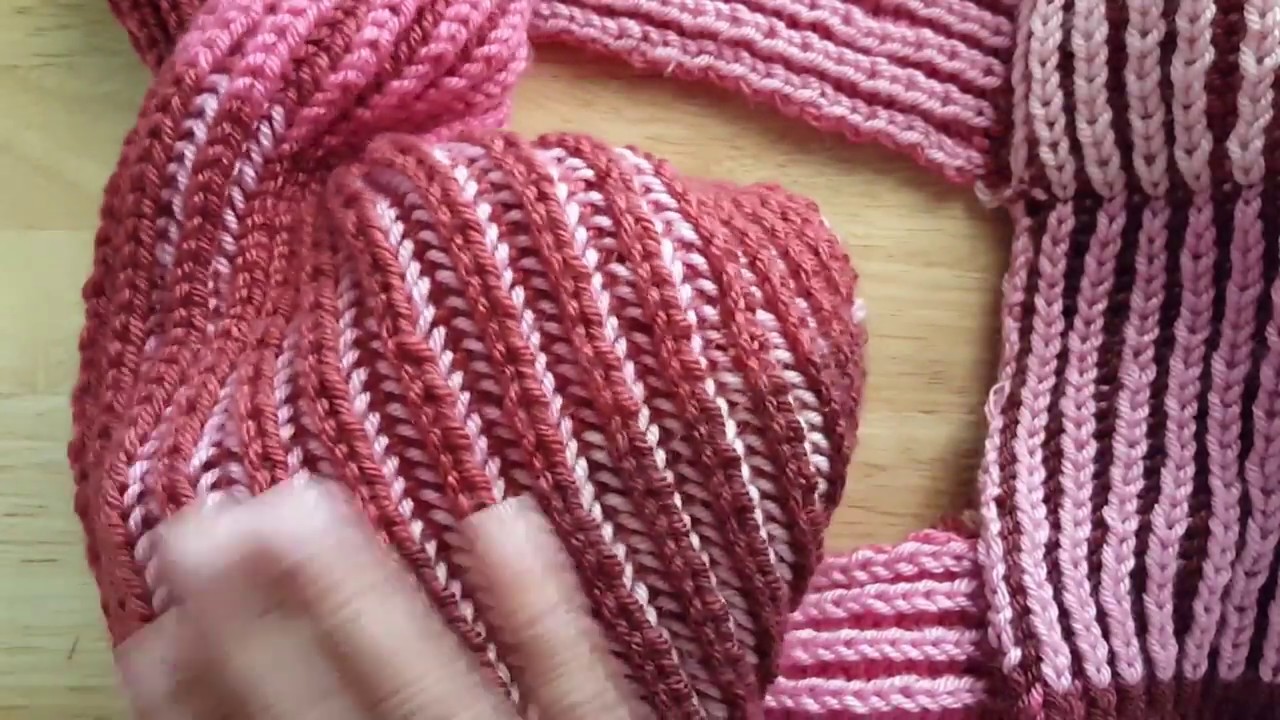The photograph captures a beautifully knit scarf draped haphazardly on a light beige wooden table. The scarf, likely crafted with a mix of crochet and knitting techniques, showcases a high-contrast pattern created by intertwining yarns of various shades — from pastel pink to hot pink, deep burgundy, and hints of red and purple. The textile curls and folds upon itself, creating a dynamic shape that extends from the center to the right, and then loops back toward the center. The right side of the scarf appears darker, perhaps due to shadows cast by softer indoor lighting, suggesting the light source is from the upper right. In the lower left corner, a light-skinned hand is partially visible but blurred in motion, adding a sense of activity and interaction with the textile. The image exudes a cozy, detailed atmosphere with its intricate knit patterns and varied color palette, emphasizing the craftsmanship involved.